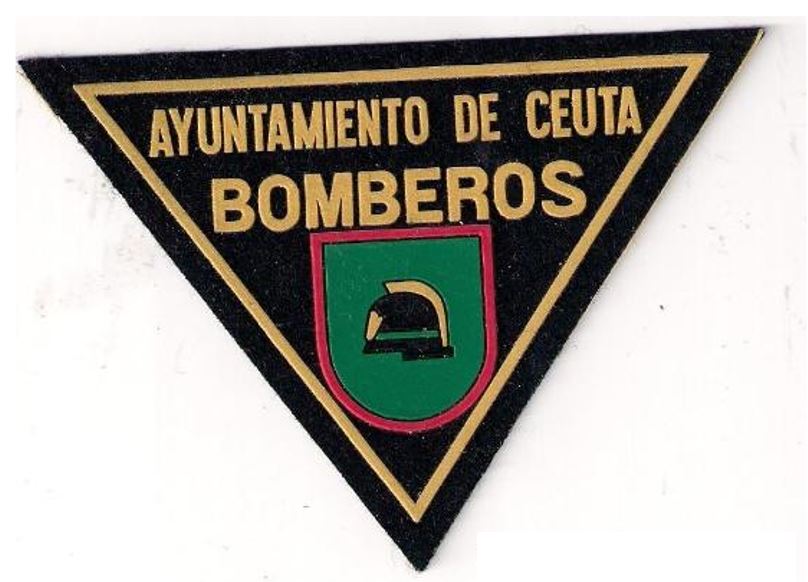The image depicts a textured patch, potentially fabric rather than a sticker, displayed against a white backdrop, possibly lying on a table or affixed to a wall. The patch is triangular in shape, with two points at the top and one point at the bottom, creating an upside-down orientation. The primary background color is black, inset with a smaller yellow triangle just inside its edges. 

Inscribed within the yellow triangle are the words "Ayuntamiento de Ceuta" on the first line and "Bomberos" on the second, indicating the text is in Spanish. Below this text is a distinctive emblem: a red-outlined shape resembling a tongue or a shirt pocket with a green interior. Central to the green area is a black helmet featuring a white stripe where the forehead would rest and a yellow emblem at the front. A definitive yellow crest or mohawk-like detail adorns the helmet, enhancing its striking appearance. This emblem denotes affiliation with the fire department ("Bomberos") in Ceuta.